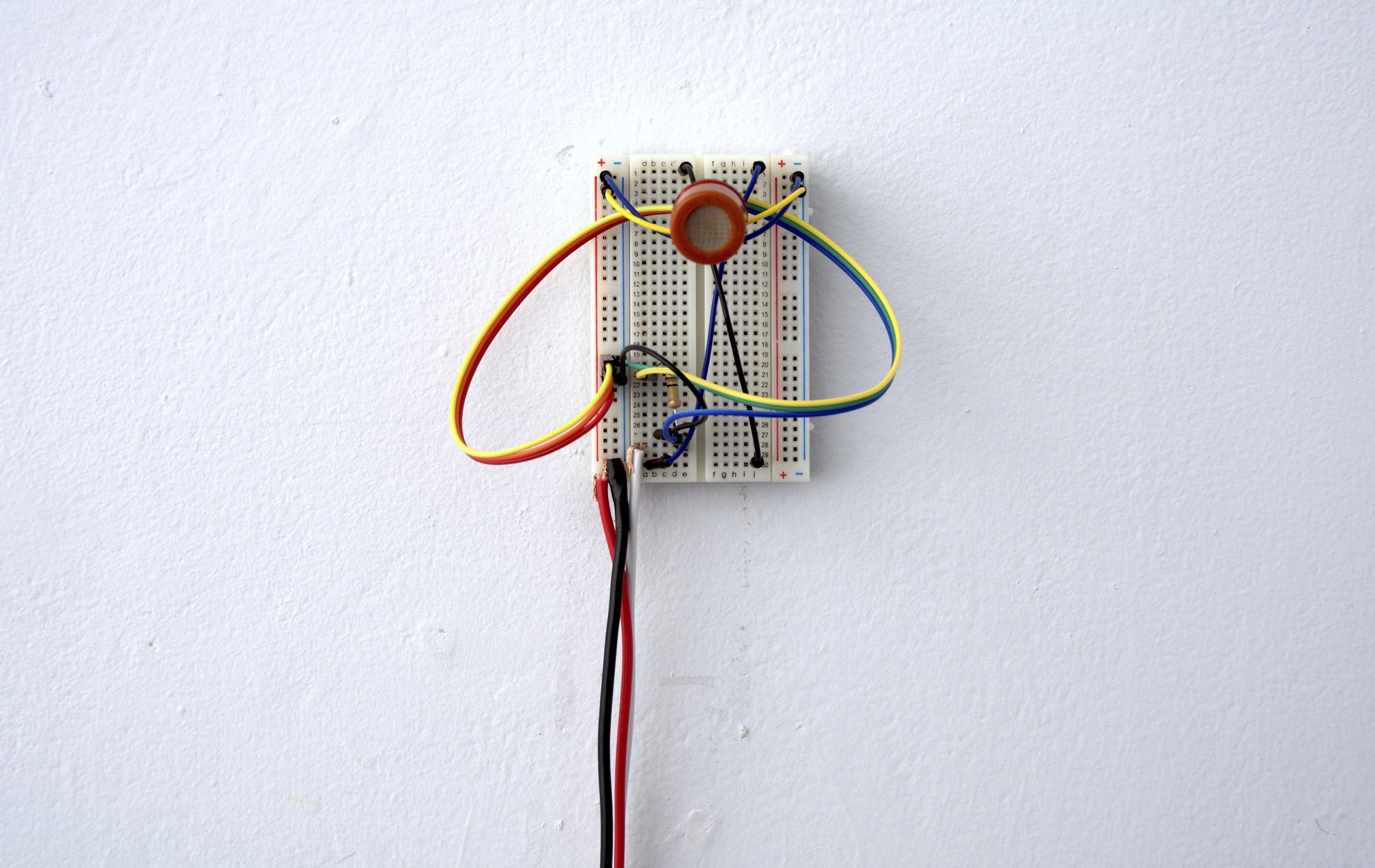The image depicts a sophisticated electrical outlet panel mounted on a white wall. The outlet, resembling a tray or pad, features numerous connection points marked with letters and numbers along the axes, indicating specific terminals for wiring connections. The panel features various colored wires plugged into designated spots: a yellow wire that bridges both a positive and a negative terminal, and a red and blue wire interconnected by a cylindrical connector, likely a wire joiner. Additionally, the bottom section holds a power source with black, red, and white wires, identifiable by their exposed copper ends making contact with the outlet dots. In the upper portion of the panel, a round knob-like object is connected with yellow and blue wires extending from each side. The panel, appearing either as plastic or white metal, includes small circular plug-in points, indicative of a detailed and specific circuitry setup designed for managing multiple electrical connections efficiently.